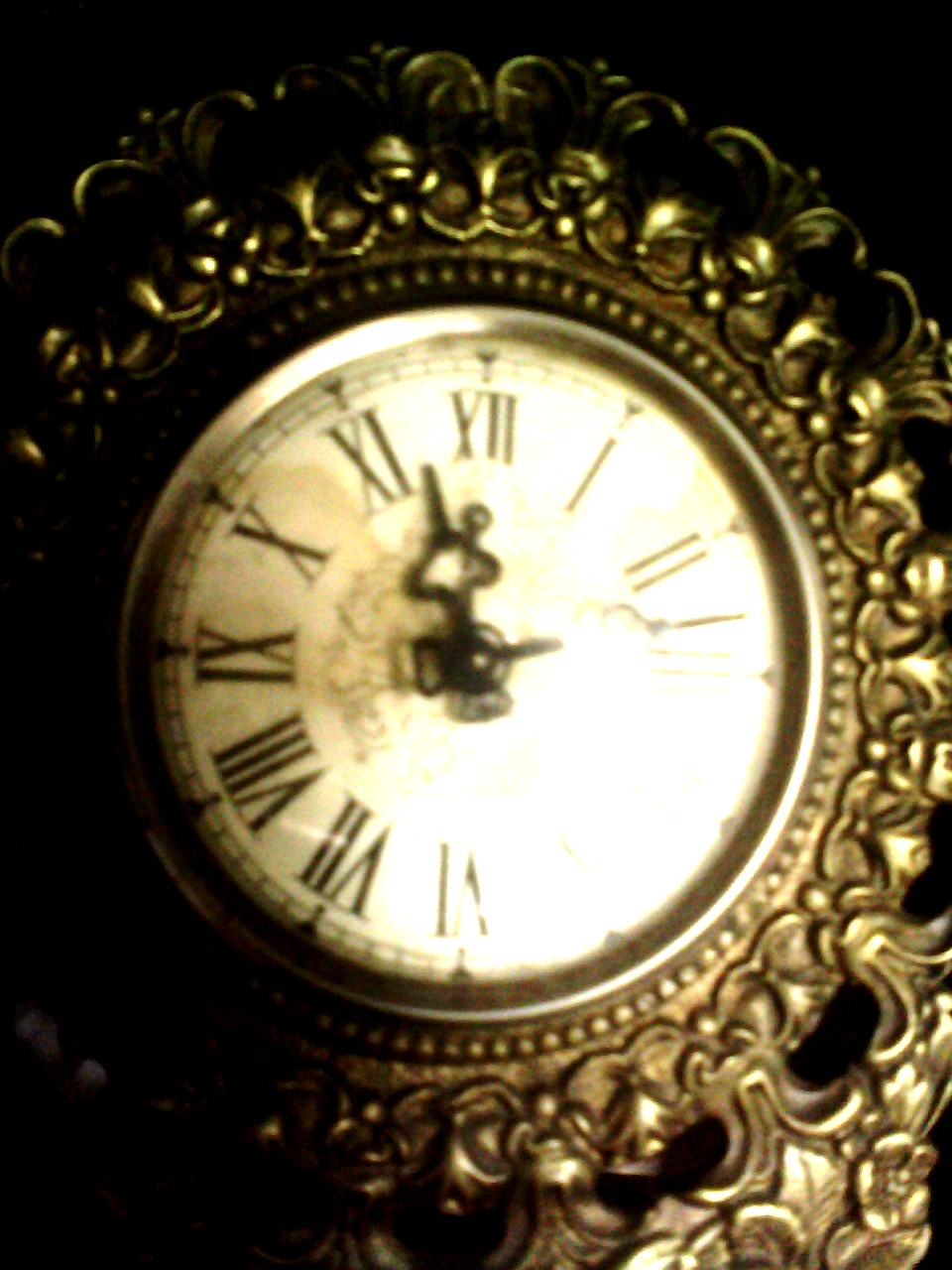This image showcases a highly ornate and detailed clock with an intricate, golden-brassy metal frame. The circular clock face is white to off-white, featuring black Roman numerals from I to XII, with XII at the top and VI at the bottom. Black hands, designed with open fancywork, display the time, which is either 11:13 or 11:15. Surrounding the clock face is a double circle of black hour and minute markers. 

The clock's frame is richly adorned with elaborate metalwork, including patterns of leaves, flowers, and other curving decorative shapes, giving it an opulent appearance. This ornate frame includes a beaded border directly around the clock face and various open sections revealing a black backdrop. The bottom right corner of the image is notably overexposed, making the fine details in that section hard to discern. Overall, the craftsmanship of the clock's frame, with its intricate and gilded florals and leaves, stands out prominently against the simplicity of the clock face.